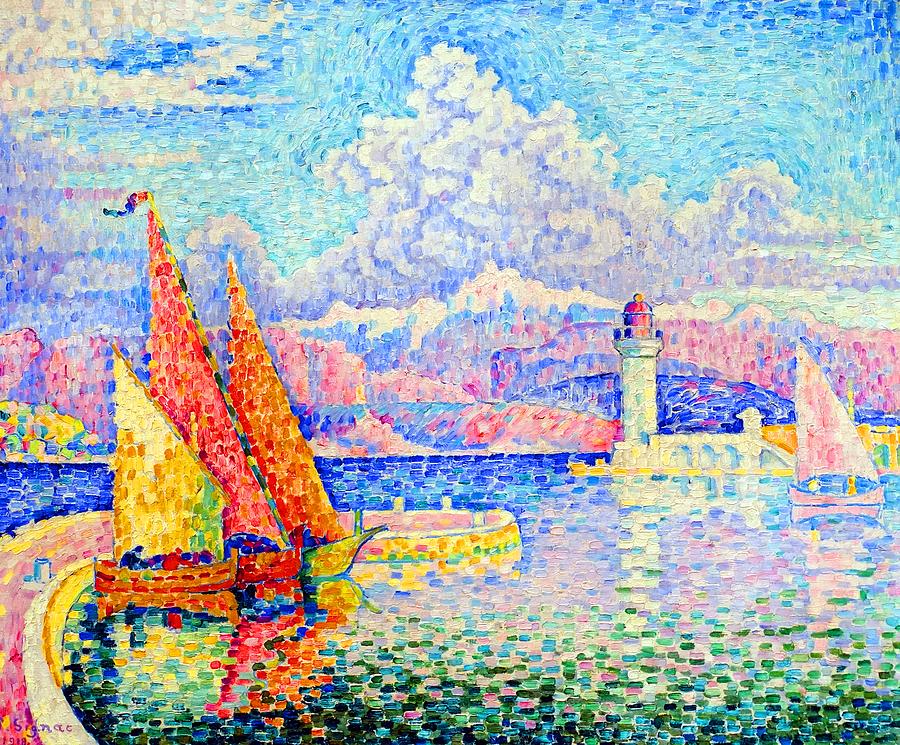This Impressionist painting vividly captures a lively marina or port scene using a striking array of colors and textured brush strokes. The composition features a visually stunning water area that transitions from the dark greens and blues at the bottom to lighter hues of blue, pink, beige, and dark blue towards the center. A green foreground gradually dissipates as it recedes into the distance. 

Nestled in the center of the canvas is a coastline, flanked by a prominent lighthouse on the right. The sky above is a medley of blue, light purple, and white, fragmented by billowing clouds. Below this dynamic skyline, a mountain range emerges in soft pink and blue tones.

On the right side of the water, a solitary sailboat floats, adding tranquility to the scene. In contrast, the left side is bustling with activity, showcasing three vibrant sailboats—painted in vivid yellows, reds, and oranges—docked along what appears to be a pier within a pink and yellow harbor area.

The artist employs thick, short, rectangular brush strokes, lending the painting a textured, almost tactile quality. These tiny, deliberate paint applications blend together to form a cohesive, dynamic image that impresses upon the viewer a richly detailed and colorful maritime panorama.